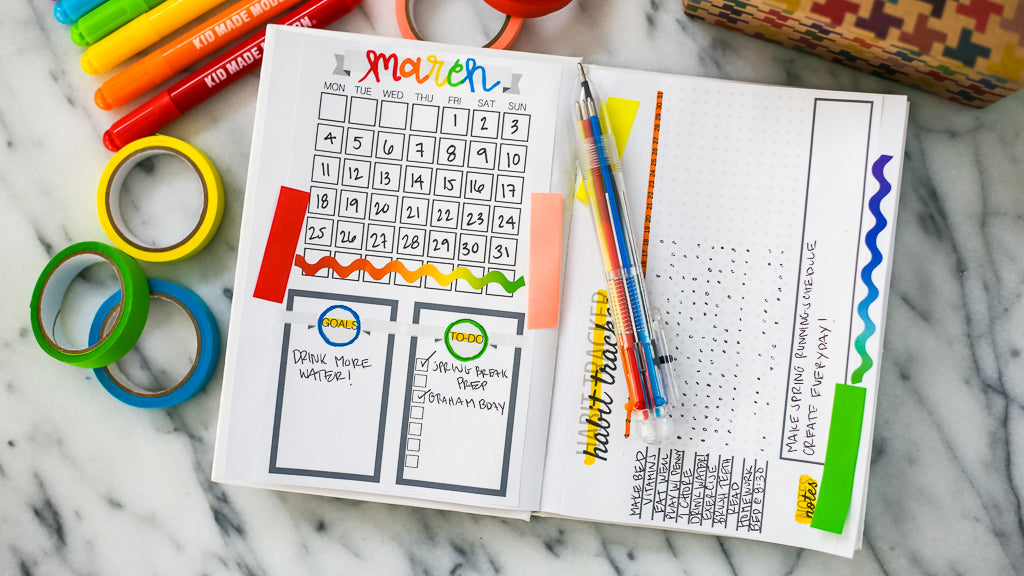The image showcases an open planner set atop a black and white marble countertop. The planner is opened to a colorful March calendar, with the month spelled out in red, orange, yellow, green, and blue letters. Dates are numbered from 1 to 31, starting with the 1st on a Friday and ending with the 31st on a Sunday. There is a notable use of multicolor elements, including a squiggly line and colorful highlights throughout the calendar. A piece of red tape and a line run through parts of the calendar.

Key features include a gold circle with "Drink more water" written inside and another section circled in green for a to-do list that includes tasks like "Spring break prep" and "Gram body." Adjacent to the calendar, on the opposite page, are sections for habit tracking and notes like "Spring running schedule" and "Create everyday."

Resting on the planner is a color-changing pen, accompanied by a set of markers in red, orange, yellow, green, and blue, all labeled with "Kids make something." Surrounding the planner are various rolls of tape: yellow, green, and blue on the left side and red and orange above the planner. The detailed organization and striking use of colors make the planner a vibrant focal point on the sleek marble surface.